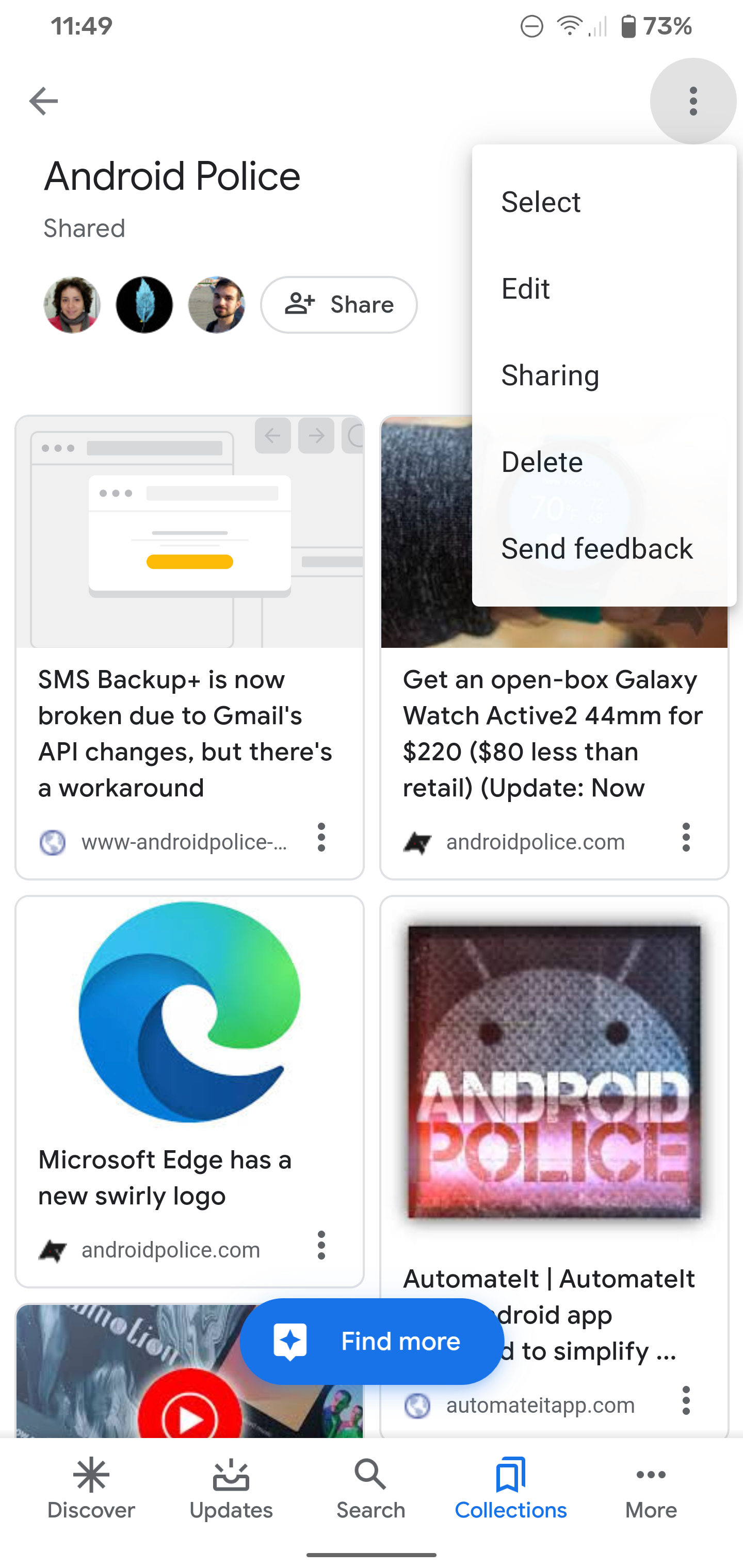The image depicts a screenshot of multiple articles from a news app. At the top, the header reads "Android Police" with the word "Shared" in grey lettering beneath it. Below the "Shared" label, there are profile pictures of different individuals, indicating shared content. The image showcases three full articles and a fourth one that is partially cut off. 

The first article, positioned at the top left, is titled "SMS Backup Plus is now broken due to Gmail's API changes, but there's a workaround." The second article, at the bottom left, is titled "Microsoft Edge has a new swirly logo." The third article, located at the top right, headlines with "Get an Openbox Galaxy Watch Active 2 for $220, $80 less than retail." The fourth article is not fully visible in the image.